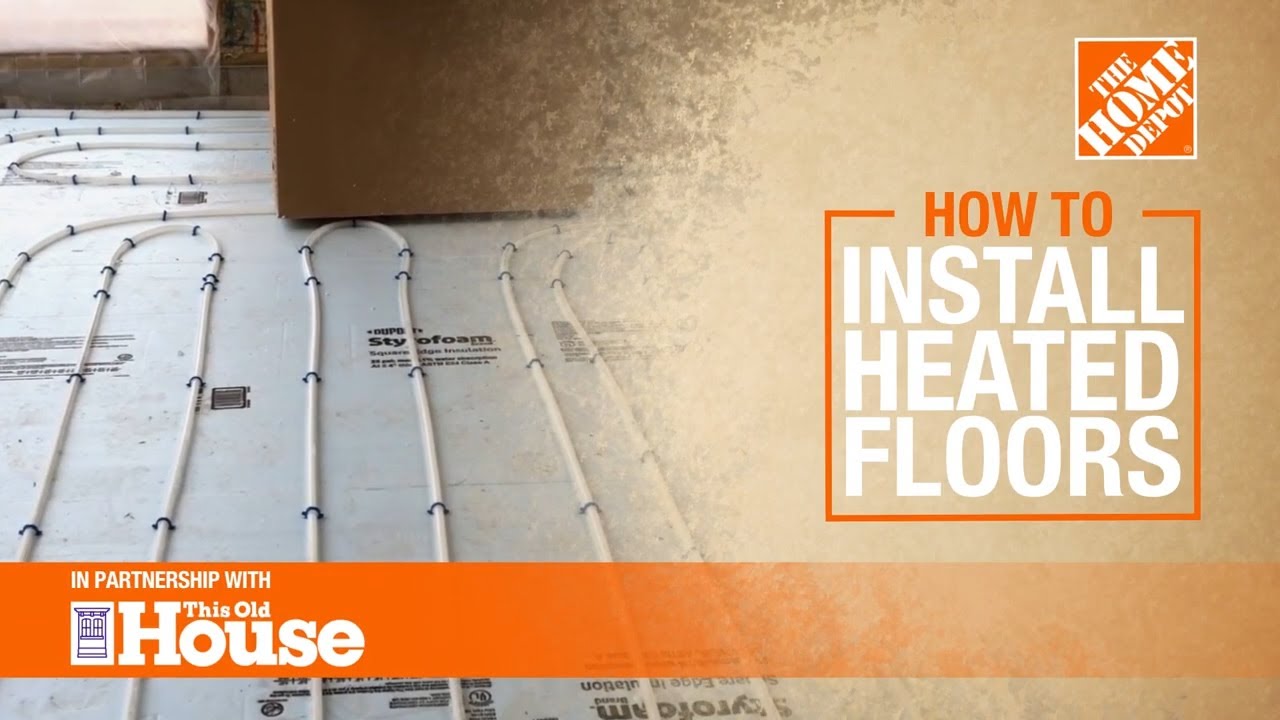The image depicts an instructional advertisement for installing heated floors. Dominating the visual, the right side features an orange square with bold text in all caps: "HOW TO" in orange and "INSTALL HEATED FLOORS" in white. Adjacent to this, in the top right corner, another orange square contains the white, diagonally placed "The Home Depot" logo. Below, an orange strip spans the width of the image, bearing the words "in partnership with This Old House," accompanied by the logo of a house on a white background in the bottom left corner. The left half of the image showcases a concrete floor with a styrofoam backing. Upon this surface, white and black heating cables are neatly arranged. Additionally, a small blue piece, possibly used to secure the cables, is visible on the floor. Text indicating "styrofoam" appears at one point to further describe the floor's material.